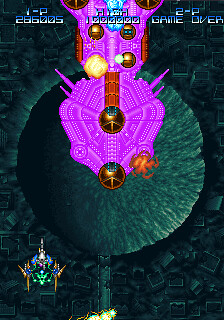In this image, we're looking at the game screen for a two-player game that has just ended, as indicated by the "Game Over" text displayed prominently. The final score achieved is 286,005, while the high score on record is 1,000,000. The game's visual setting features a massive, dark bluish crater with a concrete-like texture. This crater is detailed with a narrow, centered line reaching from its middle to the bottom edge. Surrounding the crater, various square structures can be seen, adding to the complex terrain of the game. Additionally, there is a mysterious structure or beam located towards the lower left corner of the screen, though the details remain unclear.